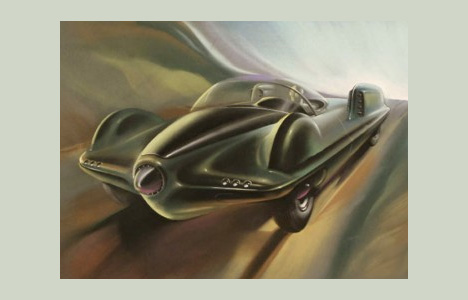The image is a digital painting of a futuristic and sleek sports car, featuring a very modern design. The car has a low, flat profile with a dark green body, seamlessly flowing into an almost conical, black front nose, resembling the front of an old airplane without the propeller. The vehicle is encased in a glass bubble-like cover, similar to a fishbowl, allowing a clear view of the off-white, mannequin-like driver inside. The painting suggests the car is speeding through an abstract landscape of dark greens, browns, and tans, blending together, with the car appearing to be in motion. The entire artwork sits on a pale green background, with an olive green border framing the piece. The wheels of the car are black and smooth, emphasizing its fast and aerodynamic design, and the car's movement is suggested by a blurred effect and impressionistic, oil-painting style.